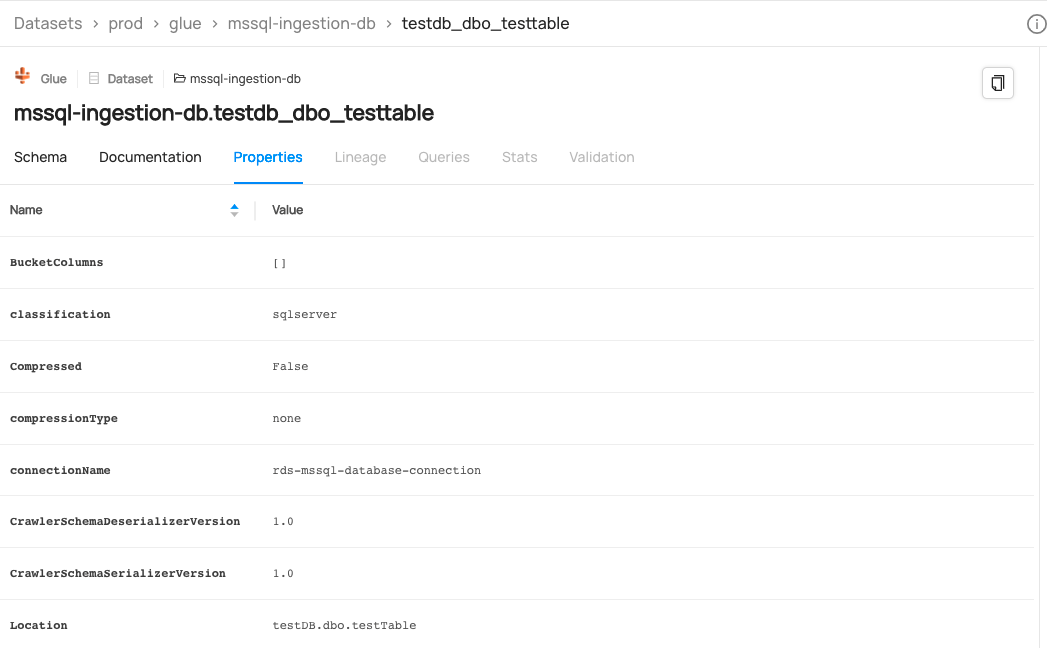This image features a predominantly white background with a gray horizontal line near the top. Beneath this gray line, the text "data sets PROD glue MSS QL-ingestion-DB test DB_DBO_testable" is displayed. Another gray line follows this text.

The image then shows an entry labeled "MSSQL-ingestion-DB.testDB_DBO_testable," which appears to be referring to a Glue dataset within some kind of data integration or ETL tool. Below this, a navigation menu offers various options including "Schema," "Documentation," "Properties," "Lineage," "Query Stats," and "Validation."

The "Properties" tab is highlighted in blue with an underscored blue line indicating selection. Under this tab, detailed property information is listed, beginning with headings "Name," "Value," "Bucket," and "Columns." The detailed properties then include specific metadata such as:

- Classification: AGL
- Server Compression: False
- Compression Type: None

This structured depiction suggests a technical interface likely used for data management, showcasing details about a specific dataset and its properties within a professional data processing environment.